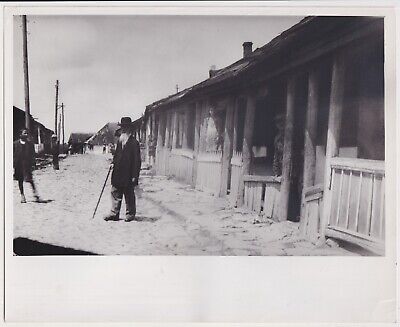This is a vintage black-and-white photograph with a solid white border, depicting a gritty scene from an old small town. The main focus is a row of dilapidated wooden buildings lining what appears to be a dirt road. The structures, which have planks missing and show signs of settling, evoke a sense of abandonment and decay. In the foreground, an elderly man with a long gray beard is seen in the distance. He is equipped with a cane and wears what resembles a modest top hat, as well as pants and shoes. The unpaved road they're standing on looks prone to turning into mud with the first sign of rain. Another figure is visible further down the road, seemingly observing the scene. Telephone poles stretch down the length of the road, suggesting some form of connectivity. The image, while grainy and a bit blurry, captures the essence of a bygone era, rich with historical ambiance.